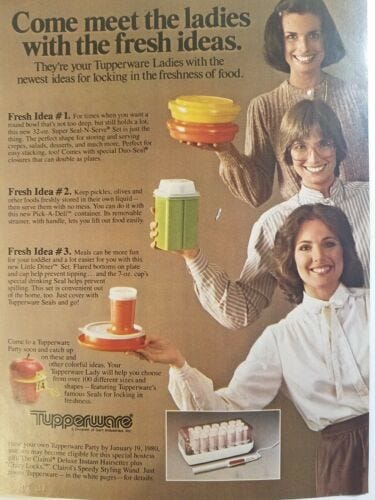This vintage magazine advertisement features Tupperware with a distinct 1970s flair. The ad is laid out in a rectangular format, with text on the left and images on the right. At the top, a bold headline invites readers to "come meet the ladies with fresh ideas," followed by a subtitle that describes them as "your Tupperware ladies with the newest ideas for locking in the freshness of food."

On the right side of the page, the same woman is superimposed three times, each instance slightly offset and overlapping with the others, giving the illusion of three different women. She appears to be in her 30s or older, with brunette hair, dressed in standard 1970s housewife attire including long-sleeve blouses and skirts or pants. She is smiling broadly in each pose, exuding happiness and confidence in the Tupperware products she holds in her right hand.

Each superimposed image of the woman is associated with a "Fresh Idea" caption on the left side, detailing versatile uses of Tupperware products. Fresh idea number one might involve using a medium-sized round bowl; idea number two could showcase a jar; and idea number three perhaps highlights a lunch plate and cup set. All these fresh ideas emphasize innovative storage solutions for keeping food fresh.

At the bottom right, the recognizable Tupperware logo is accompanied by what might be a set of electric hair curlers, suggesting how the ladies achieve their styled hair. The overall feel of the advertisement is nostalgic, aiming to encapsulate the excitement and practicality of Tupperware products in the 1970s.